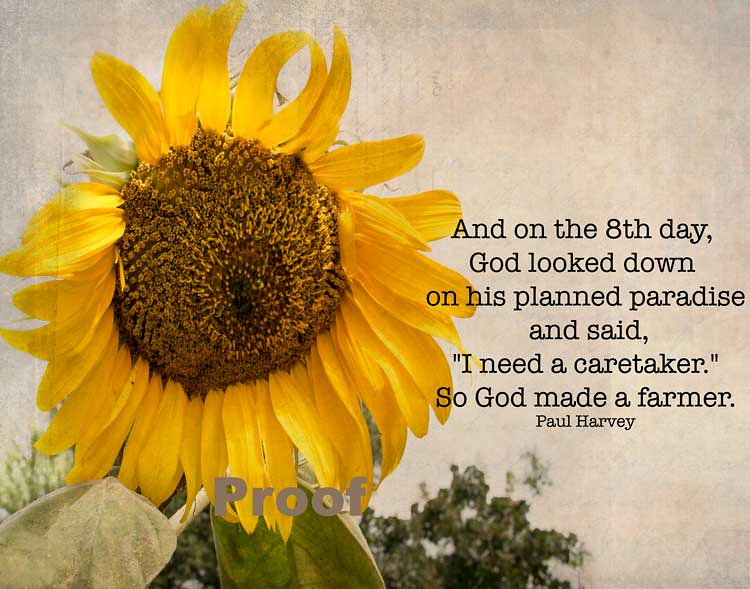This is a large square poster featuring a prominent, slightly worn-out sunflower occupying most of the left side from top to bottom. Below the sunflower, a large green leaf hangs down, surrounded by smaller, fine green leaves. The sunflower appears to have aged, suggesting it has seen many days of sunlight.

In the background, there is a textured blend of brown and gray, giving the image an aged, almost rustic feel. Across the bottom of the sunflower, the word "PROOF" is displayed in gray, uppercase letters.

On the right side of the image, there is centered text that reads:
"And on the eighth day, God looked down on His planned paradise and said, 'I need a caretaker,' so God made a farmer."
This inspirational quote is attributed to Paul Harvey, whose name appears in smaller black text underneath.

Overall, the image combines elements of nature and a heartfelt message, creating a sense of nostalgia and appreciation for farmers.